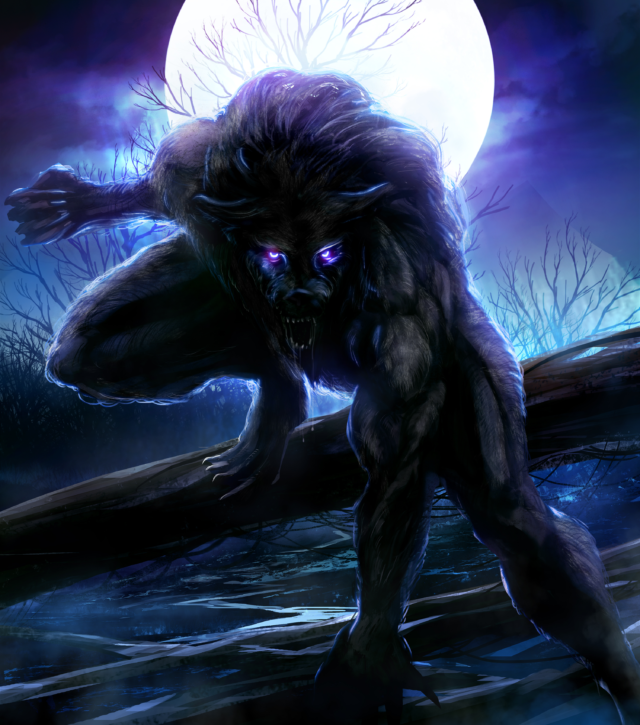The image portrays a menacing, comic book-style illustration of a werewolf, shown in a single panel with dark, purple hues. The werewolf stands crouched on a horizontally fallen tree trunk, creating a foreboding stance with one muscular leg raised on the log while the other is stretched out in a ready position. Its left hand is planted firmly on the ground while its unnaturally thick right hand is cocked back, poised for action. With fur slicked back and bathed in deep shadows, the creature's eyes glow eerily white with a touch of purple and blue, its open mouth revealing sharp teeth. The backdrop features a bright full moon glowing against a blue and purple sky, casting a ghostly light on stark, leafless tree branches that stretch ominously into the night. The overall effect is haunting, with the werewolf's piercing gaze and shadowy details heightened by the contrasting moonlight, underscoring a deep sense of unease and terror.